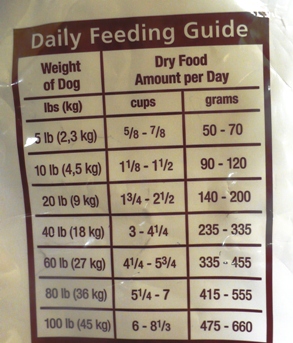This image captures a detailed label from a bag of dog food. At the top of the label, there is a graph titled "Daily Feeding Guide." The graph is divided into columns; the first column lists the weight of the dog in both pounds and kilograms, while the second column indicates the recommended amount of dry food to feed per day based on the dog's weight. For instance, a dog weighing 10 pounds (4.5 kilograms) should be fed between 1 1/8 to 1 1/2 cups of food per day, which is equivalent to 90 to 120 grams. The guide covers a range of weights from 5 pounds to 100 pounds, providing specific feeding amounts to ensure that dogs receive proper nutrition according to their weight.